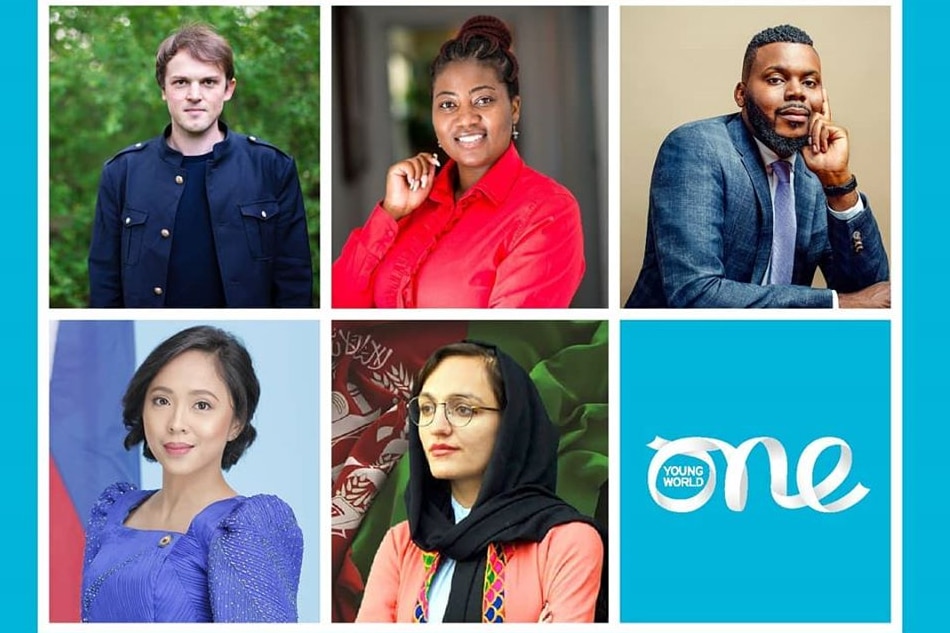The image is a composite of five headshots arranged in a grid format, each bordered by a crisp white background, which creates a delineated grid of white matrices. The remainder of the webpage features a light turquoise blue hue framing the grid on the left and right sides. Notably, the bottom right segment of the grid does not contain a headshot but displays the numeral "1" formed with ribbon-like text including the phrase "Young World" inside the “O.”

- The top left headshot showcases a young man clad in a black jacket over a black t-shirt, posed against a lush green outdoor background.
- Adjacent to him, on the right, is a woman dressed in a hot salmon blouse, captured indoors.
- The next headshot to the right features a young man in formal attire with a suit, thoughtful with his chin resting on his left hand.

Moving down to the bottom row:

- The bottom left image presents a young woman in a purple dress against a vibrant, colorful background.
- In the middle of the bottom row is a young woman wearing a headscarf and a pink cardigan, standing before a patterned backdrop.

This carefully arranged collection of headshots, complete with detailed attire and backgrounds, highlights the individuals alongside the distinctive "Young World" logo, enveloped by the serene turquoise blue of the website.